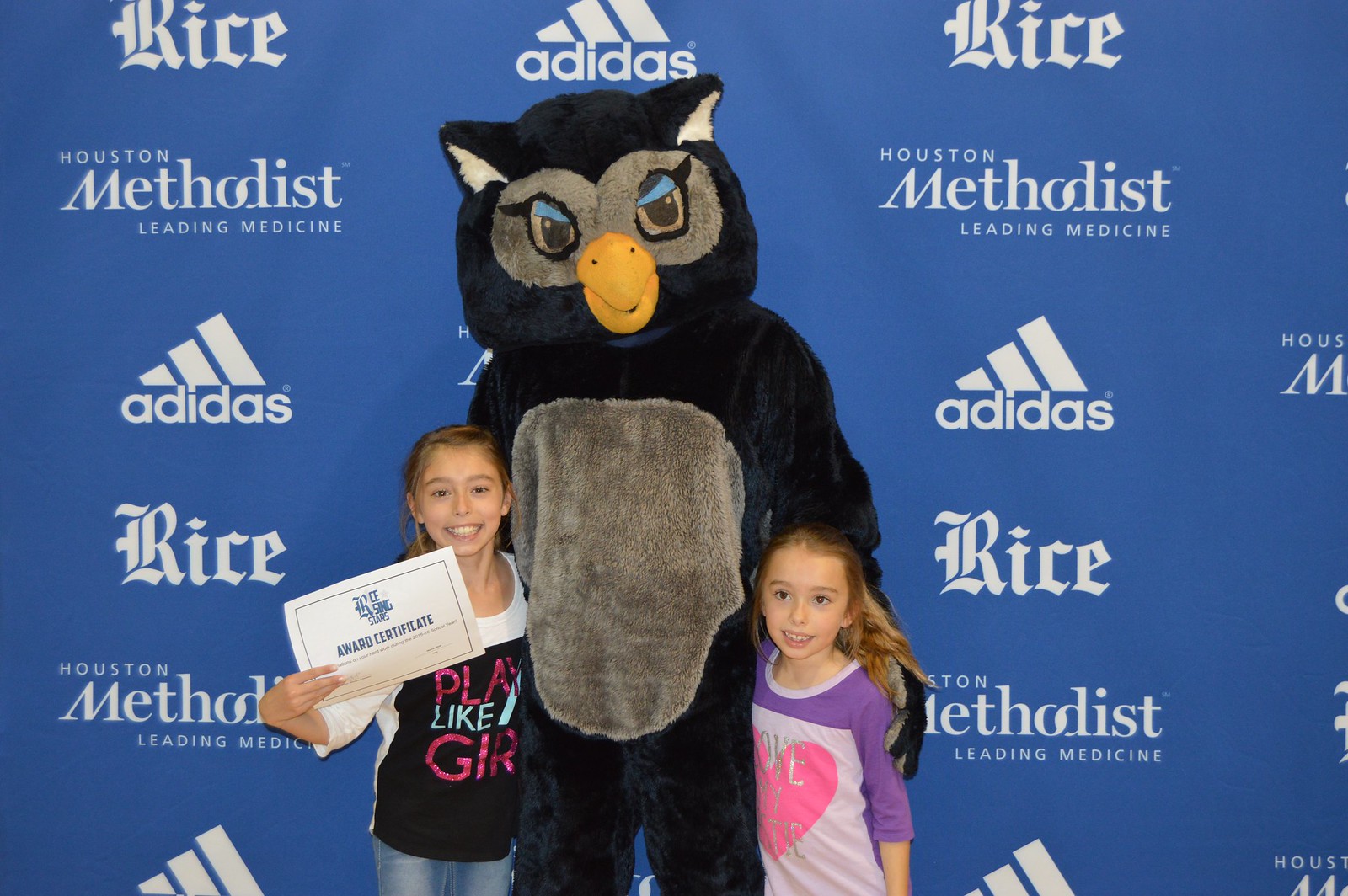In this photograph, two young, blonde girls of elementary school age are standing on either side of a person in an elaborate owl mascot costume. The owl mascot features a black suit with white inside its ears, a large yellow beak, and a gray belly. Its eyes are accentuated with gray fur and blue eyelashes. The older girl, positioned on the left, is likely in first to fourth grade and is proudly holding an award certificate that reads "Rising Stars." She is dressed in a black t-shirt that says "Play Like a Girl." The younger girl on the right, slightly shorter, is wearing a purple, long-sleeve t-shirt with writing that includes the word "love." Both girls are smiling brightly. Behind them is a blue banner adorned with multiple white logos, including Houston Methodist Leading Medicine, Adidas, and Rice.